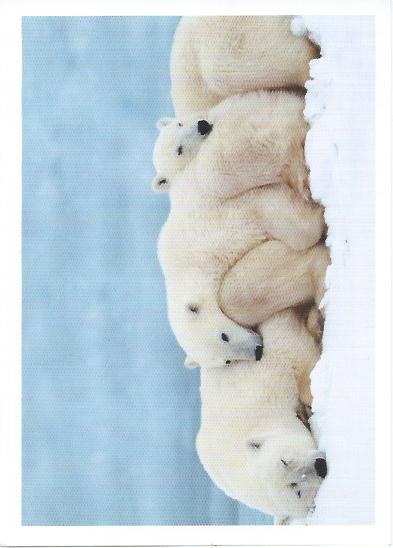This image, positioned as if a postcard turned 90 degrees counterclockwise, depicts three polar bears nestled together on a snowy surface. The trio of bears appear intertwined, with the landscape rotated so that the ground lays vertically on the right and the sky on the left. The leftmost bear faces toward the viewer, its black nose and partially open eyes visible, resting its body fully on the snow. The central bear angles left, its head laying on the thigh of the bear behind it. The rightmost bear faces right, seemingly asleep with its head cushioned on the knee of the center bear. In the backdrop, a choppy, blue-gray scene suggests an overcast sky or potentially shaded, distant snow. Horizontal scan lines run across the image, adding a textured, scanned effect. The polar bears, predominantly white with hints of light brown, showcase their dark eyes, noses, and the inner parts of their ears, underscoring their gentle rest in a cold, serene setting.